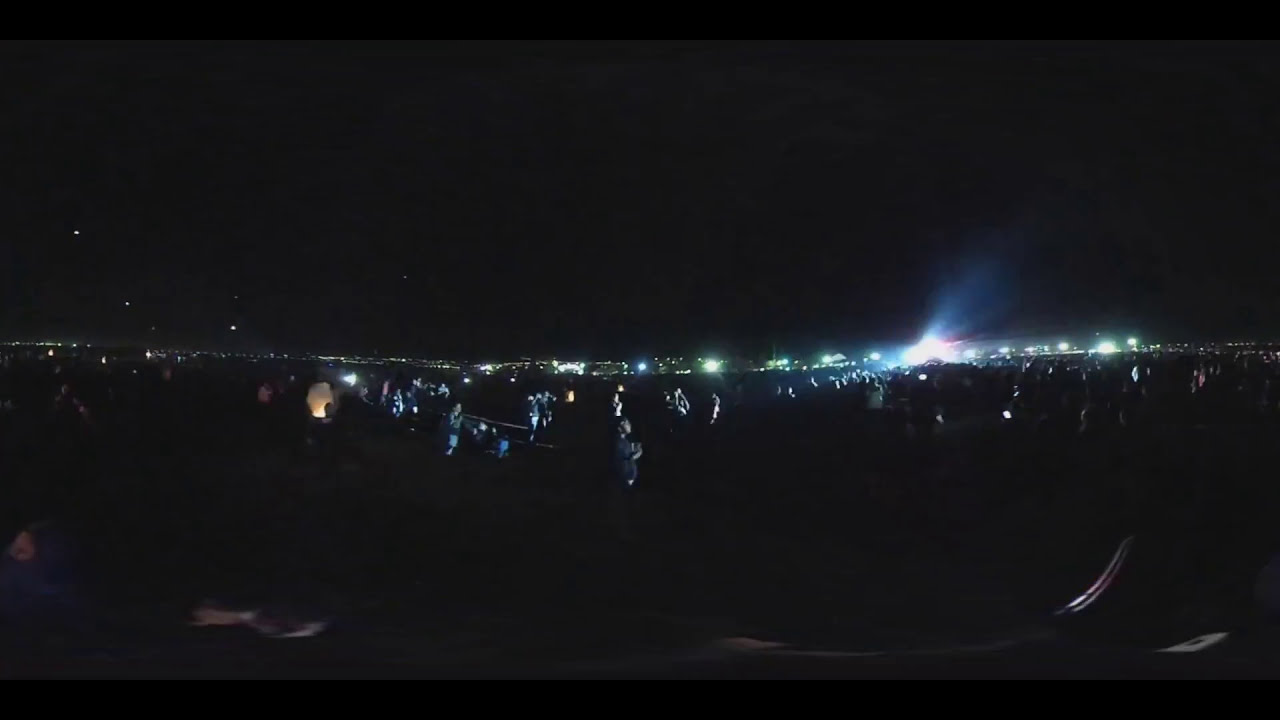The image captures a nighttime outdoor event, set against a pitch-black sky devoid of stars or the moon. In the foreground, there are several indistinct shapes and blurry shadows. Numerous people are standing in a field, mostly facing to the right, as if they are looking up at a show or performance. Scattered small lights from personal flashlights faintly illuminate some individuals. Near the center of the image, a strong beam of light suggests the location of a stage or focal point. In the background, a series of brighter lights near the horizon creates a horizontal line, possibly from a faraway city skyline or an array of buildings. The overall scene is dark, with only 4 or 5 small specks of light in the sky, adding to the mysterious atmosphere.